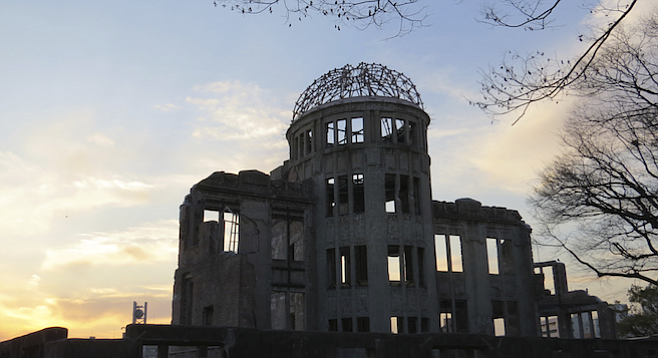The image captures a large, multi-level building that appears to be either in the process of construction or ruin. The structure is predominantly made of concrete or stone with a white-brick appearance on the walls. A prominent central tower with an open wire mesh dome made of interlocking steel beams stands out. Surrounding the tower are numerous archways that form multiple windows, some of which are open to the elements while others reflect the sky, suggesting the presence of glass.

Extending from the left and right sides of the building are additional walls with similar arch windows. At the rear, a large wall nearly as tall as the central tower looms. In the background, a sunset or sunrise with some clouds creates a dramatic lighting effect, casting the building in a silhouette. The outline of bare trees to the right of the image hints that the scene was captured in winter or early in the year, adding to the somber and mysterious atmosphere.